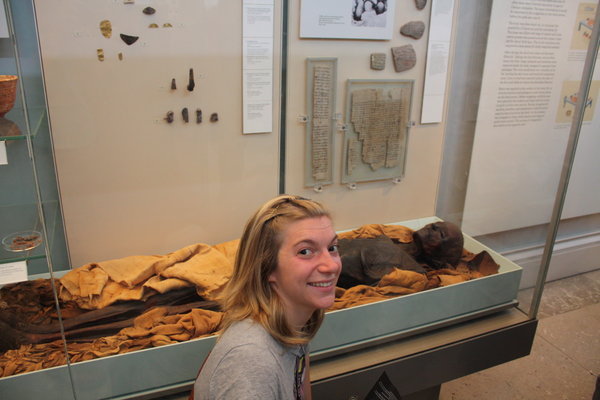A young woman, likely in her late teens or early twenties, is pictured sitting very close to a glass-enclosed display in a museum. She has shoulder-length blonde hair and dark-colored eyes, and she is smiling broadly, revealing her teeth. She is wearing a gray t-shirt featuring the Rolling Stones lips logo. The display next to her contains an exceptionally tall Egyptian mummy, which appears fossilized or calcified, with visible blackened skin around the ribcage and lower legs. The mummy rests in a dark-colored, low white box lined with a gold-colored cloth that partially covers its midsection. Behind her, the museum wall features various artifacts, informative write-ups, and diagrams detailing the interior of a pyramid.